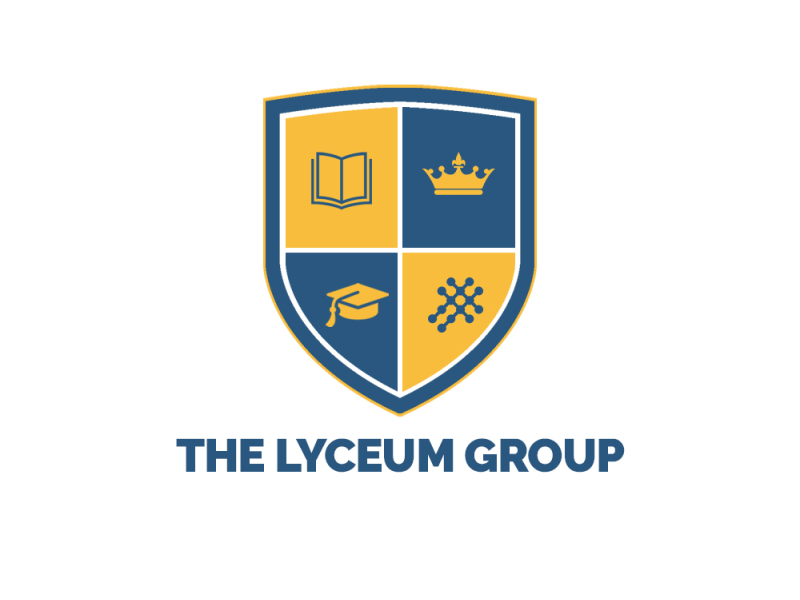The image depicts the logo of the Lyceum Group, which is designed with detailed iconography and colors to represent various elements. The logo features the group name, "Lyceum Group," written in dark blue text at the bottom. Above the text is a shield with a layered border: starting with a yellow outer border, followed by a blue border, and an inner white border. The shield is segmented into four quadrants, each displaying a distinct symbol. 

The top left quadrant has a yellow background featuring the silhouette of an open book in black. The top right quadrant displays a yellow crown against a blue background. The bottom left quadrant shows a yellow graduation cap (mortarboard) on a blue background, with the tassel draped over the left side. The bottom right quadrant has a yellow background with a blue geometric design: two intersecting lines forming an 'X' shape, with a circle (or bulb) at each of the four endpoints.

The overall color scheme predominantly includes shades of blue and yellow, creating a cohesive and striking visual representation of the group's identity.